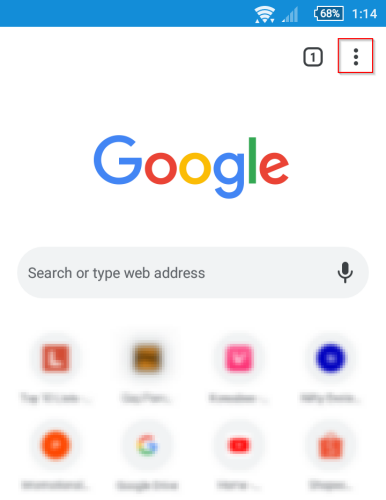The screenshot captures the Google.com homepage on a mobile device. At the top of the screenshot, a blue status bar displays essential information including Wi-Fi signal strength, battery level, mobile connection bars, and the current time (1:14). Directly below this status bar, there are three vertical dots indicating the settings menu for Google, and a black box with the number '1' inside it is positioned to the left.

Centrally placed is the iconic Google logo, featuring its distinctive colors: blue G, red O, yellow O, blue G, green L, and a red E. Below the logo, a search bar is prominently displayed with a microphone icon to the right, allowing users to perform voice searches.

Further down the screen are two rows of four blurred bookmarks or app icons. In the first row, from left to right, there is a red box with the letter 'L', a yellow box with black text, a pink box with the letter 'V', and a blue circle containing a smaller white circle. In the second row, the sequence includes an orange circle with a smaller white circle, the Google 'G' icon, the YouTube symbol (a white circle with a red play button), and a white circle with a pink shopping bag icon.